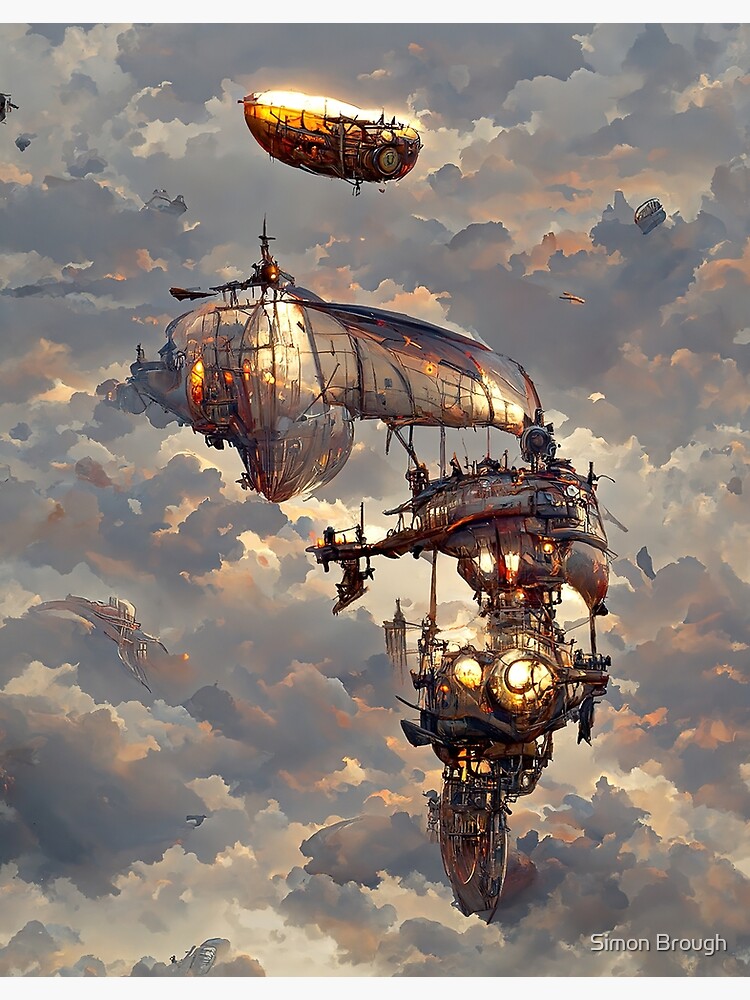This artwork by Simon Brough features a surreal, futuristic scene set against a backdrop of cumulus clouds in varying shades of white, light gray, and dark gray. Dominating the foreground is a complex, ancient spaceship-like structure, composed of multiple sections including a top segment that appears disconnected. This structure has elements resembling bicycle wheels, semi-circular vantage points, and what might be mechanisms or lights. 

Near the top center of the image, a strange boat-like object with shield-like circles and oar-reminiscent features further adds to the futuristic aesthetic. Emanating from the uppermost section of this object is a bright light. To the upper right, there is a small, difficult-to-identify item, and hovering toward the lower left is another structure that vaguely resembles a bird. Scattered across the cloudy expanse are small orange shapes that punctuate the otherwise muted color palette.

The name of the artist, "Simon Brough," is distinctly displayed in block letters in the lower right corner of the image.